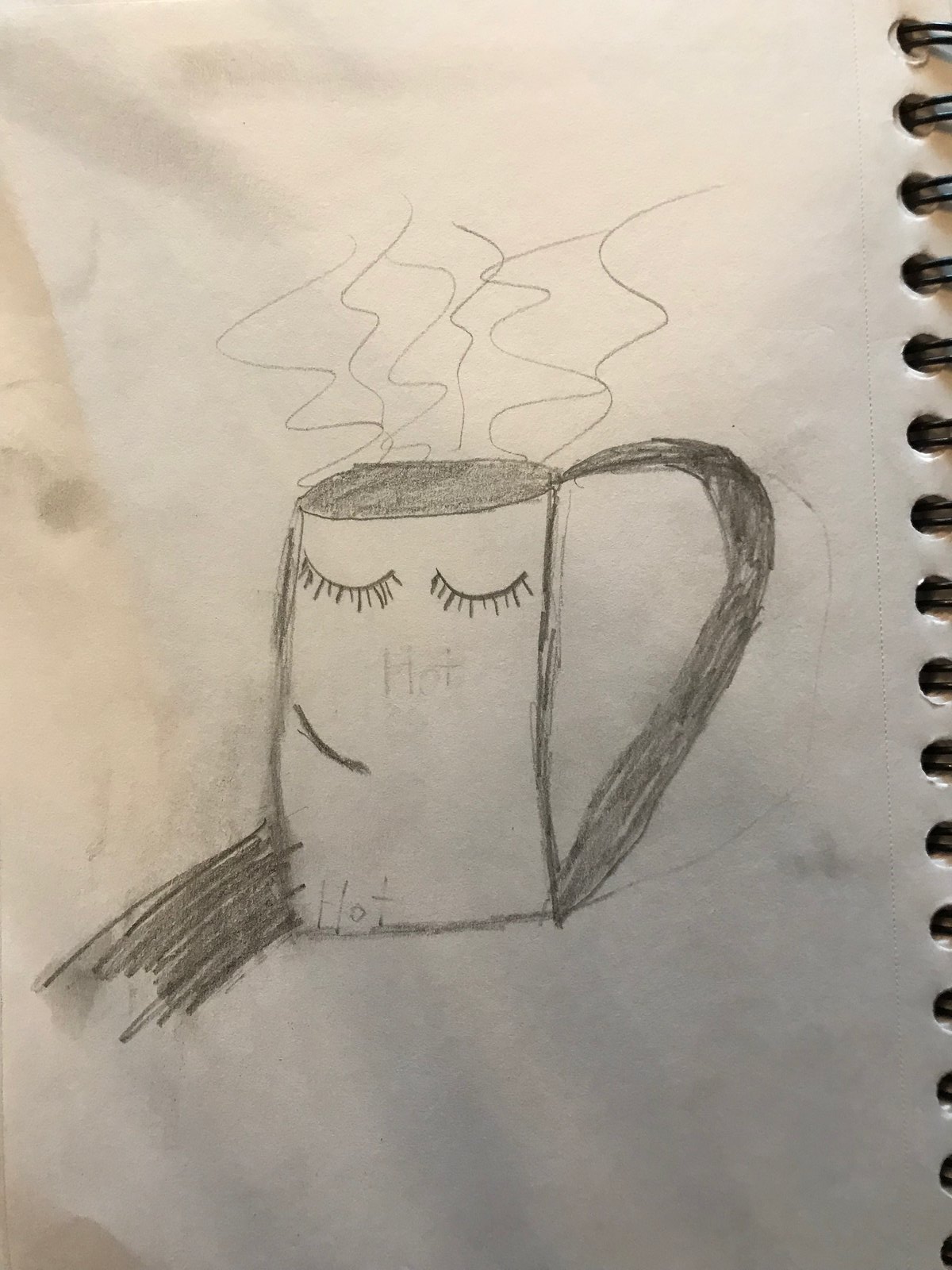This detailed color photograph features a crude pencil drawing on slightly greyish-white notebook paper, with visible spiral rings along the right edge. The main subject is a cylindrical, vertical coffee cup with a prominent, curved handle resembling half a valentine heart extending down its right side. The cup, penciled in dark grey, is characterized by its closed eyes adorned with lashes, giving it a sleepy expression, and a small, half-smiling mouth slightly tilted to the left. Squiggly lines rise from the top of the mug, indicating steam from the dark-colored liquid inside. Although there are faint, erased markings of the word "hot" near the eyelashes, they add to the sketch's charm. Beige shading on the left and greyer shadows at the bottom suggest the photograph's slight color. A circular smudge, possibly a fingerprint, is noticeable near the cup's top-left edge. Off to the left, beneath the cup, is a diagonal scribble that appears unrelated to the main drawing. The paper itself shows signs of crumpling, adding texture to the background.